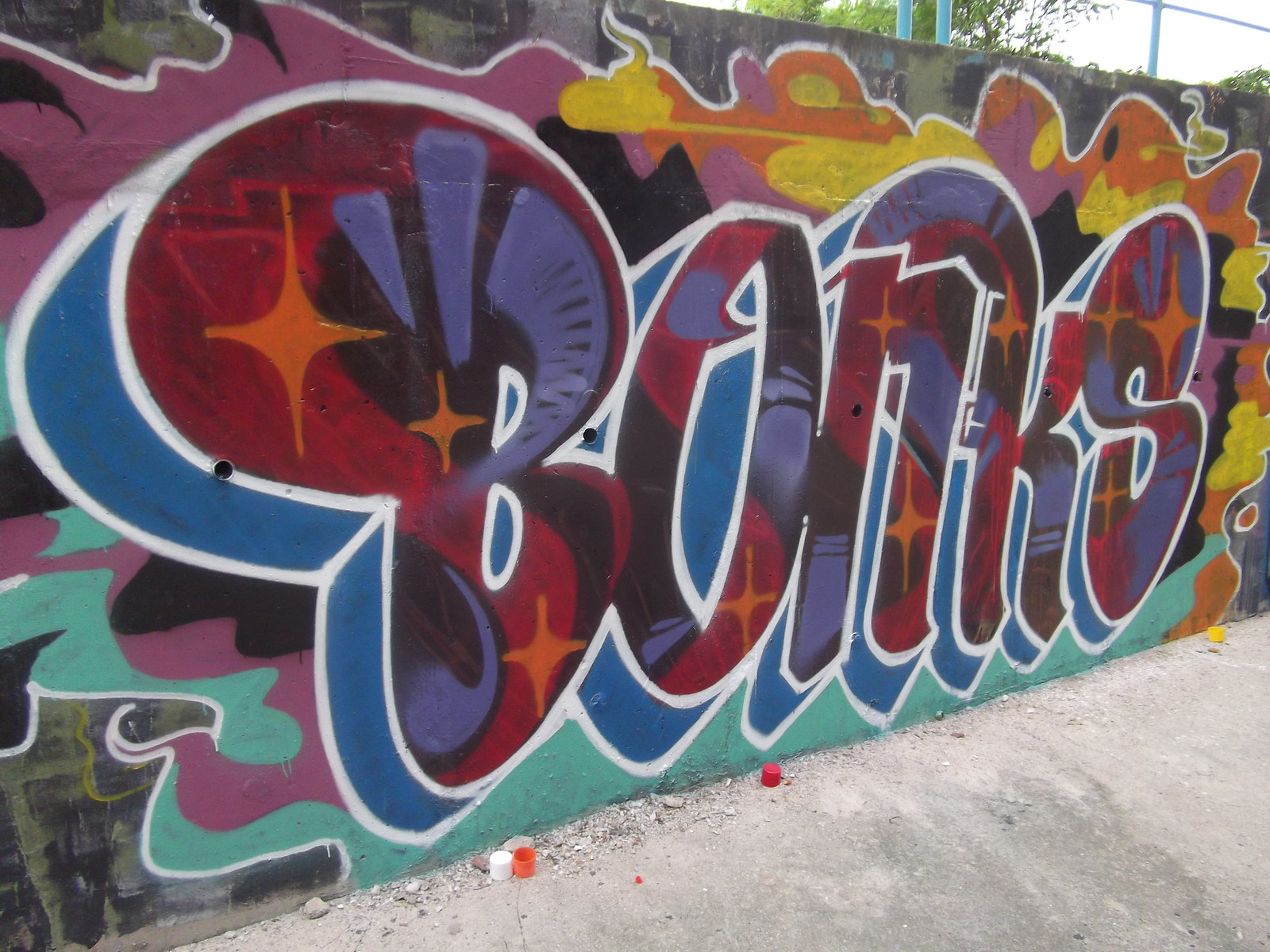The image showcases a large cement wall adorned with graffiti depicting the word "Bonks" in stylized, three-dimensional bubble letters. These letters are an amalgamation of vibrant red, blue, and white, accented with shiny orange highlights. Emerging from the letters are flames in shades of purple, orange, and yellow, adding a dynamic flair to the artwork. In front of the wall lies a cement ground, scattered with various spray paint caps, including colors such as yellow, pink, peach, white, red, and orange. The wall, potentially part of a public park, features several pipes and holes. Above the wall, a light blue handrail is supported by several pillars, and a white sky with a backdrop of greenery completes the scene.